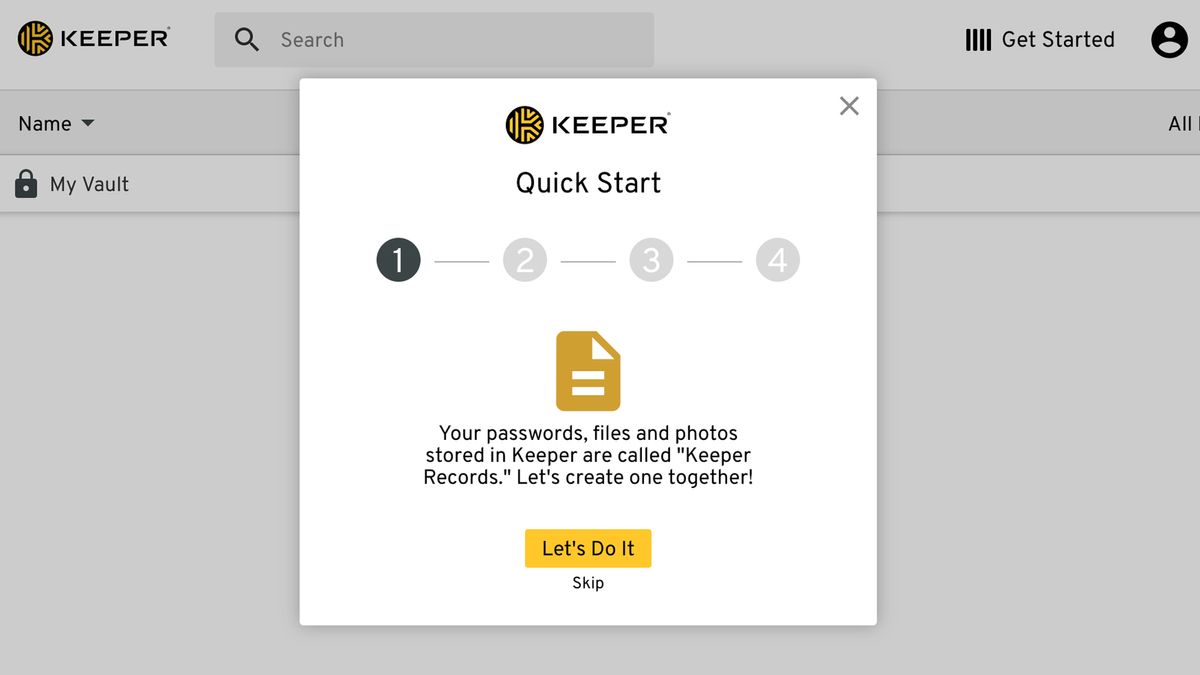This screenshot captures the interface of the desktop version of the Website Keeper. Dominating the background is the main layout of the website, featuring the prominent Website Keeper logo, a black circle adorned with alternating black and yellow stripes. Adjacent to the logo sits an empty search bar, and to its right, a series of tools are displayed under the heading "Get Started," suggesting options for new users to create a profile. In the upper-right corner, a profile icon indicates the option for users to log in or create a new account. 

Superimposed over the website background is a dialogue box that likely appears upon a user's first visit to the site. This dialogue box, branded with the Keeper logo and labeled "Quick Start," outlines a streamlined, four-step guide for new users. The first step is highlighted and features a yellow icon with a page, accompanied by the instruction: "Your passwords, files, and photos stored in Keeper are called 'Keeper Records.' Let's create one together." Below this message are two buttons: "Let's Do It," which initiates the creation of a Keeper Record, and "Skip," for users who wish to bypass the tutorial. 

The overall aesthetic suggests a user-friendly, introductory experience designed to guide new users through the initial setup of their Keeper account seamlessly.